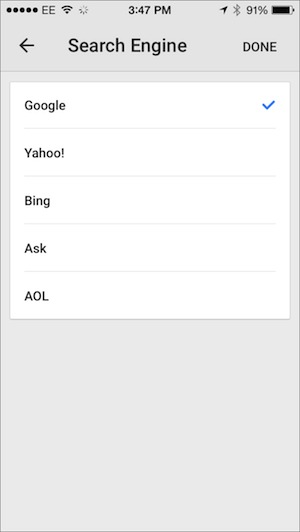The image depicts a smartphone interface for selecting a default search engine. The background is light grey, while the search engine selection area in the center has a white background. At the top of the image, the title "Search Engine" is prominently displayed in black text. To the top left, there is a back button represented by a black arrow pointing to the left, and on the top right, the word "Done" is also displayed in black text.

The interface presents a list of five search engines, each accompanied by a radio button for selection. The list is as follows:
1. Google (highlighted with a blue checkmark to indicate it is currently selected)
2. Yahoo
3. Bing
4. Ask
5. AOL

Each search engine name is positioned on the left side of the list, with the corresponding selection indicator on the right. This setup allows users to choose their preferred default search engine, which will be employed in their browser without the need to select it every time they perform a search.